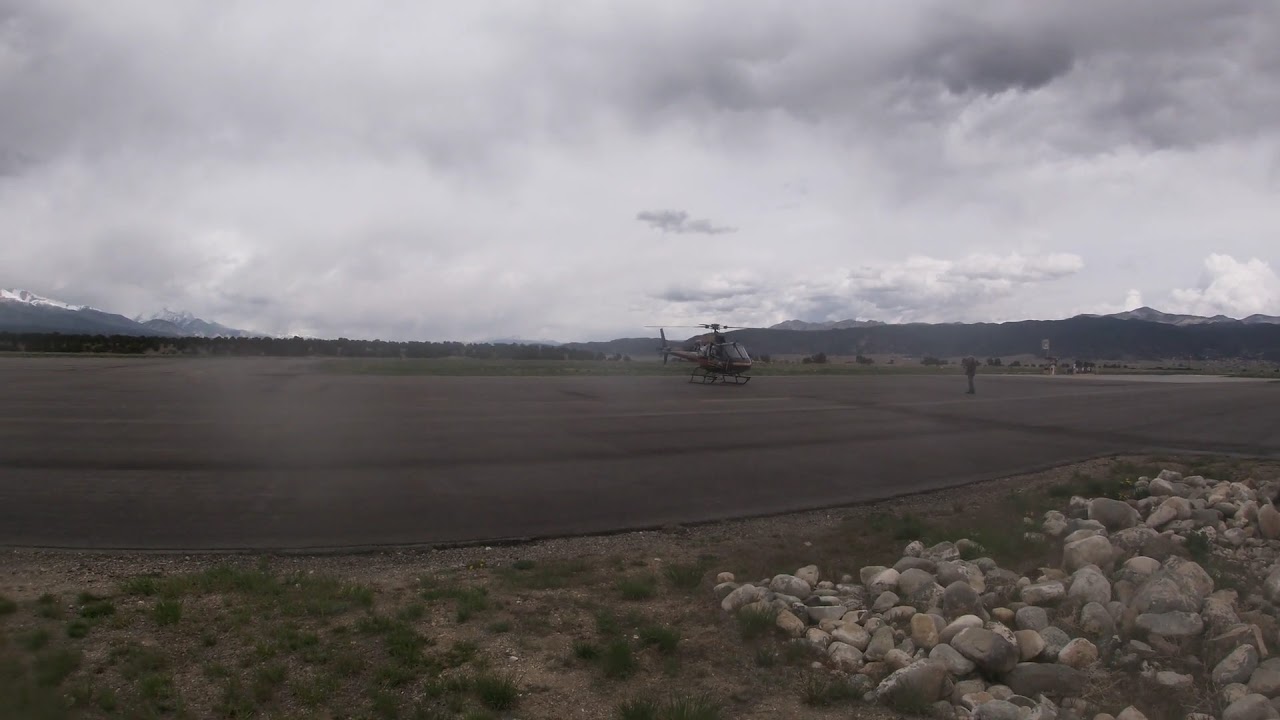In the center of the image, a helicopter rests on a brown, patchy field, its blurred propellers hinting at motion. The expansive landscape is dotted with short grass and distinctive, round-shaped stones of brown and gray hues, predominantly in the lower right corner. A man is seen walking toward the helicopter, adding a human element to the scene. The foreground features a sizable landing pad marked by clear lines dividing the field. On the left, more vegetation sprinkles the brown soil, while a nearby road and an unclear sign complete the setting. In the background, a range of majestic, snowy mountains rises against a grayish-white sky filled with clouds, creating a breathtakingly serene yet dynamic backdrop.